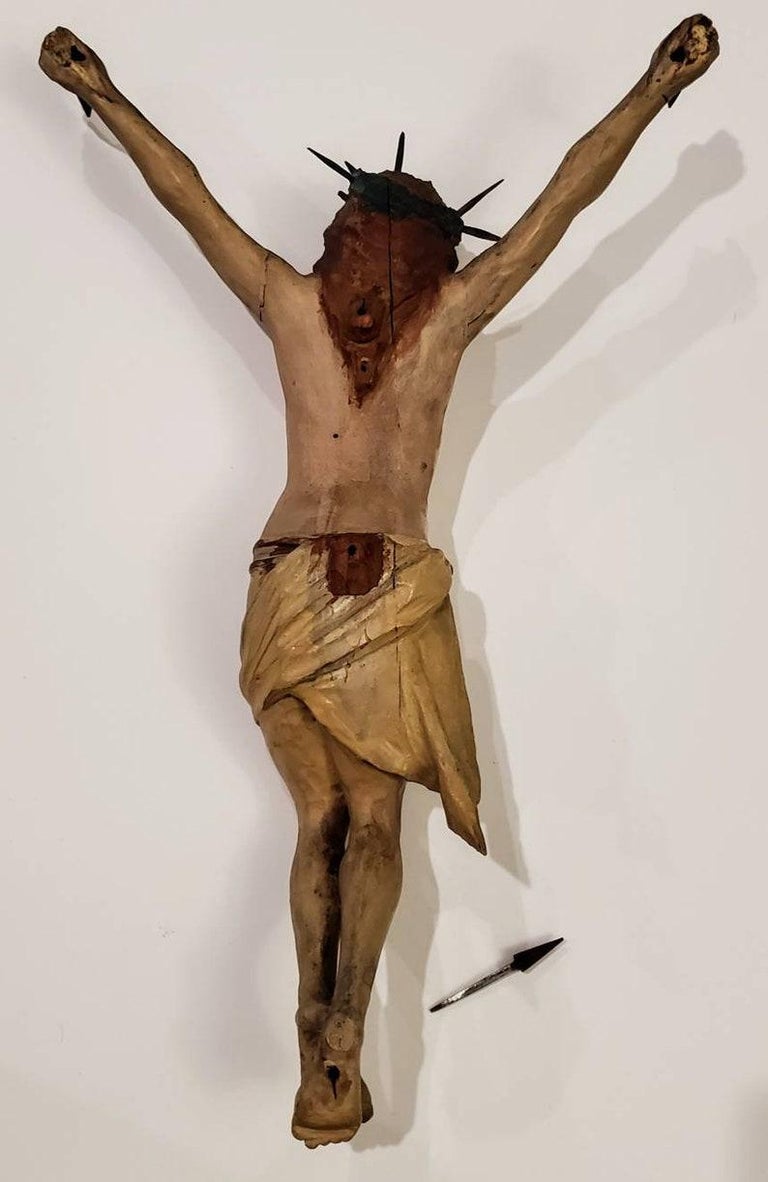The photograph depicts a detailed statue of Jesus Christ, positioned face down against a white or beige background. The statue resembles a portrayal of Christ as he was on the cross, but without the actual cross. He is only clothed with a tan material wrapped around his waist, which has a blood-stained area at the top, resembling a clasp or belt buckle. Christ's arms are outstretched wide and upward, with visible black marks in his palms indicating where he was nailed. His hair, reddish-brown and medium length, falls between his shoulder blades, and he wears a crown of thorns. The bare legs of the statue are dirty and bound together, with the ankles appearing crossed and the feet pierced by a single spike. Additionally, there is a small sideways spear located near his feet on the right side of the image, which might symbolize the spear used to pierce his side. The overall setting and posture vividly capture the crucifixion scene from a rear perspective.